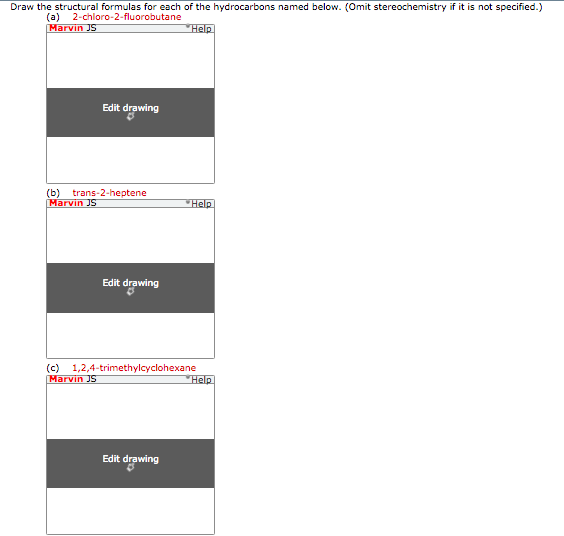The image depicts an online chemistry exercise interface where users are instructed to draw structural formulas for specified hydrocarbons. The task is to illustrate each hydrocarbon, with a particular note to omit stereochemistry if it is not specified. 

The interface includes white, blank canvas boxes designated for users to create their structural drawings. There is an "Edit Drawing" button, possibly intended for adding lines, bonds, and bond angles to the designated areas. The user's name, "MarvinJS," is visible on the interface. 

The three hydrocarbons that need to be drawn are:
1. Trans-2-heptene
2. 1,2,4-trimethylcyclohexane 
3. Another similarly complex organic compound

This chemistry exercise seems to require a comprehensive understanding of organic chemistry to accurately draw the structural formulas of these named hydrocarbons.